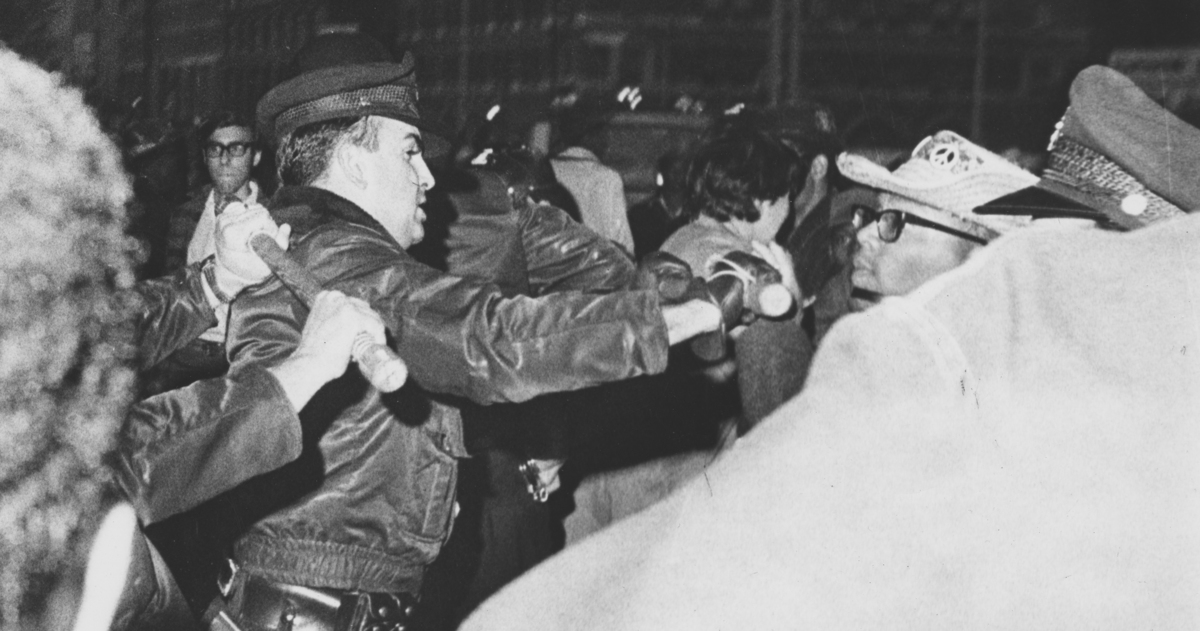This black-and-white vintage photograph, taken during the 1968-1970 Detroit racial justice civil rights protests, captures a tense encounter between police and protesters. The scene is set at night, emphasizing the stark contrasts in the image's black, white, and gray tones. On the left side of the landscape-oriented frame, a white police officer, identifiable by his hat and leather jacket, stands in profile holding up a stick or baton as if to block or fend off the crowd. The officer's assertive posture contrasts with the composed yet defiant stance of the protesters on the right, who have their hands raised. Among the protesters, the distinct figures include a black man and a white woman with her back to the camera, suggesting the diverse makeup of the civil rights movement. The background reveals a partially visible crowd, adding depth and context to the charged atmosphere. This representational and realistic photograph poignantly captures the intensity and significance of the civil rights struggle during a critical era in American history.